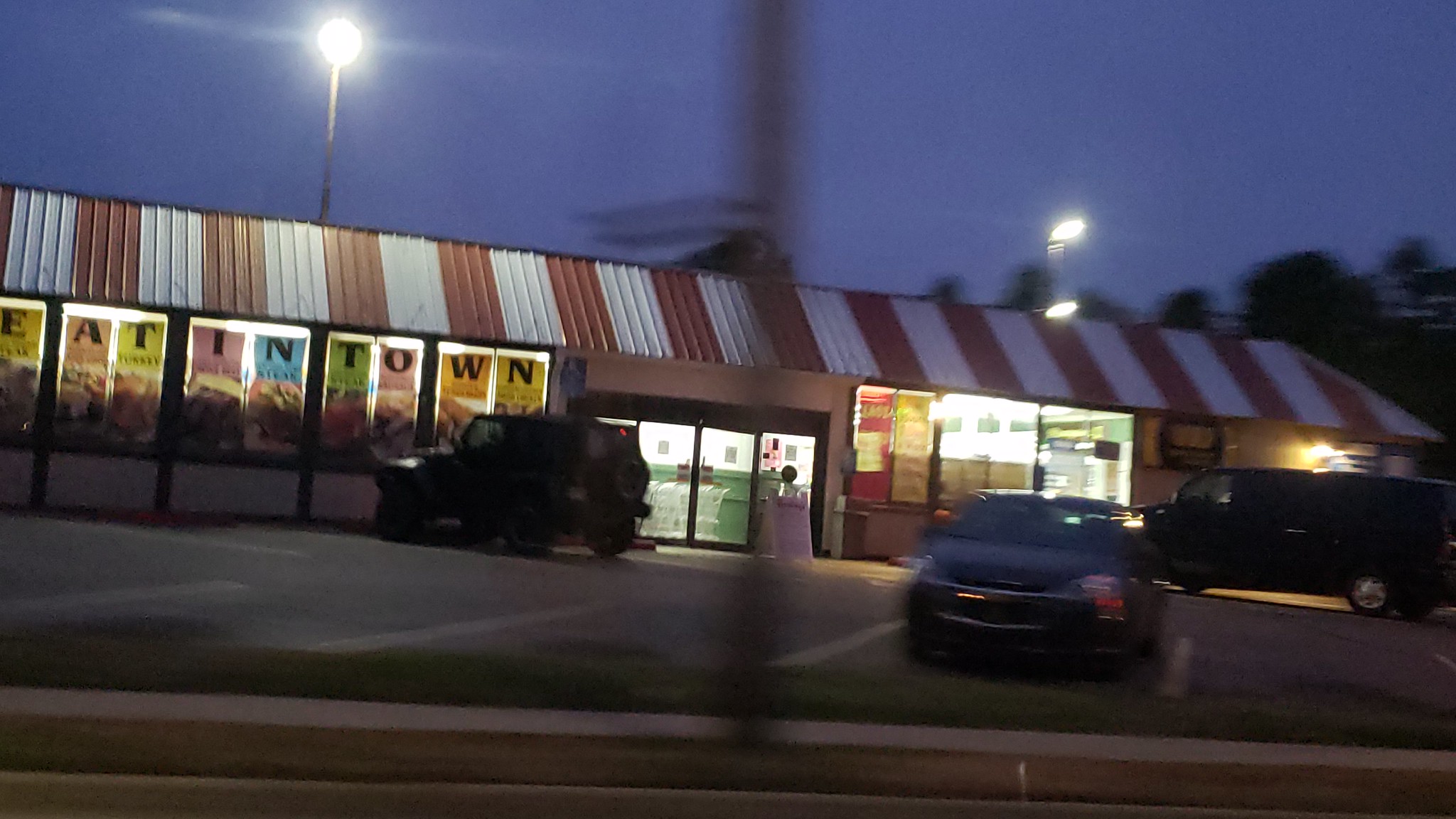This photograph, seemingly taken from a moving car at dusk, captures a long building front illuminated by two street lights positioned at either end. The sky is transitioning from dusk to full darkness, creating a dim ambiance. The building features a distinctive red and white vertically-striped metal roof. A pitched roof with what looks like a plume of smoke rising is faintly visible in the background, further adding to the scene.

The front of the building is lined with numerous windows, each displaying colorful signs that collectively spell out "eat in town," with each letter in a different colored box—yellow, brown, purple, and blue. These signs stand out vividly against the otherwise muted colors of the night.

Beneath the windows lies a row of vehicles in the angled parking lot. Closest to the left entrance, there is a jeep, followed by a dark-colored van further down on the right, and another dark-colored car parked directly across from the entrance doors. The black-framed double doors at the front of the building appear to be closed, and a curb runs along the edge of the street.

The interior lights of the store are on, casting a soft glow through the windows, and a sign is positioned directly in front of the main entrance, adding to the sense of welcome and activity within the store. Trees are visible in the distance at the end of the building, adding a touch of natural contrast to the urban setting.